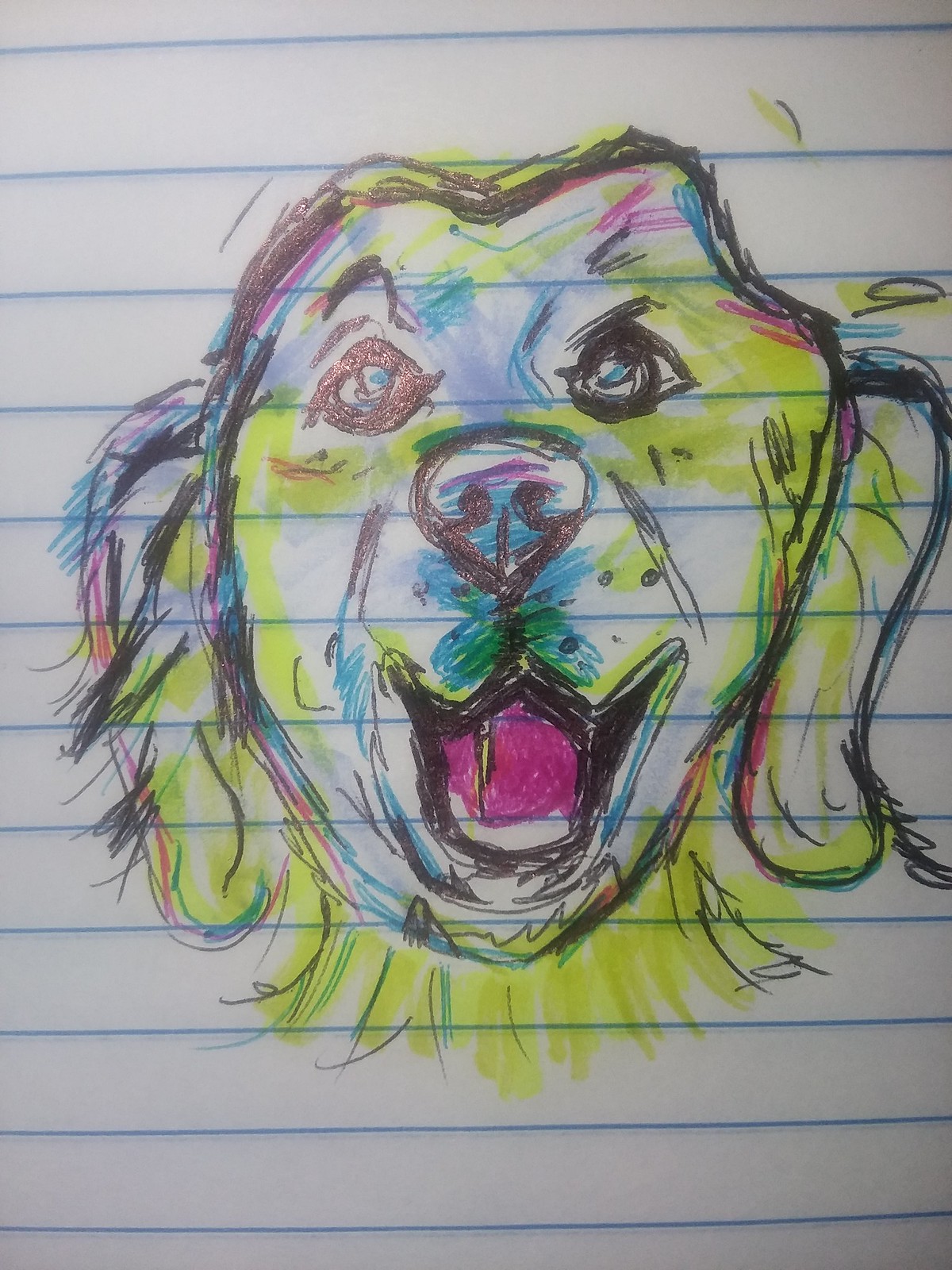This vibrant color photograph captures a detailed sketch of a dog's head, drawn on a piece of white, lined notebook paper. The paper features thin blue lines running horizontally at a slight angle. The dog's head dominates the frame, meticulously outlined in black ballpoint pen, illustrating its mouth, nose, eyes, face, ears, and part of its neck. The sketch is enriched with bright yellow highlighter, adding lively shading to the face. Additional shading and highlights are executed with a thin blue pen around the eyes, nose, and mouth. Green highlighter accents appear beneath the dog's nose and on the sides of its face, adding whimsical touches. The dog's blue eyes pop vividly, and its open mouth reveals a cheerful pink tongue, bringing an animated and expressive quality to the sketch.